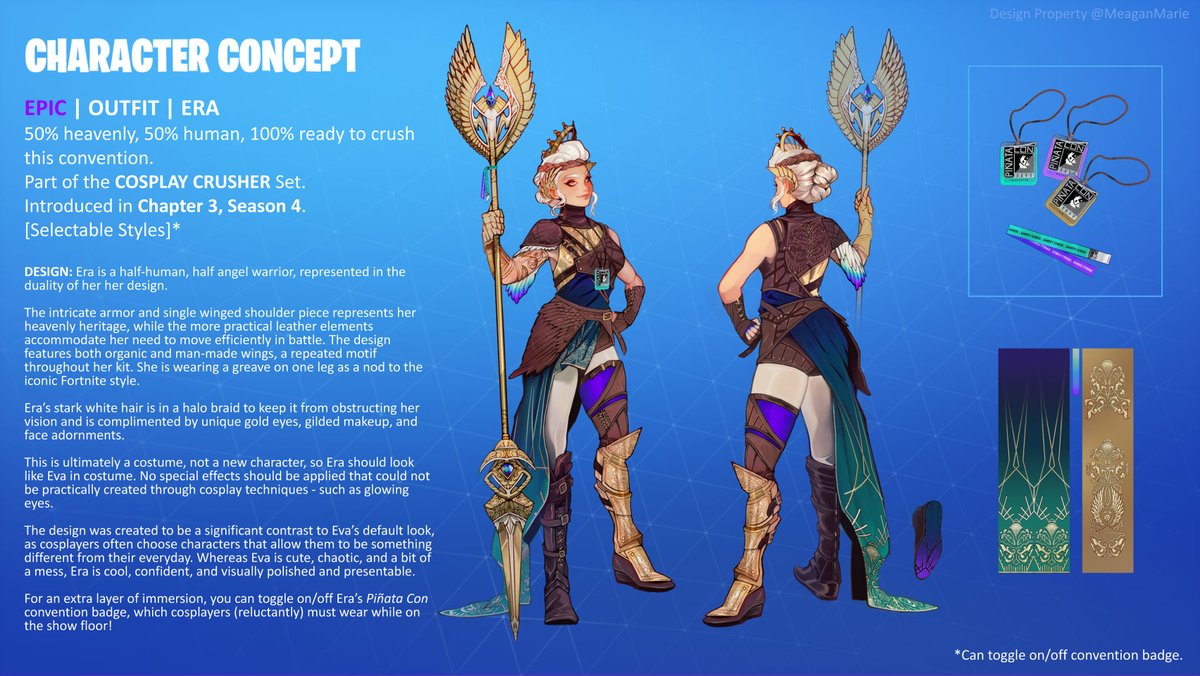The image features a detailed drawing of a female character designed for a video game, shown from both the front and back. She is depicted as a half-human, half-heavenly warrior adorned with a crown-like tiara and long, flowing white hair pulled back into a ponytail. Clad in a short brown leather tunic with a mismatched pair of boots—one dark brown leather and the other gold—the character embodies a harmonious blend of myth and fantasy. She wields a giant staff with wings and a dragon head at the top, culminating in a spear-like point at the bottom.

The background showcases a gradient from light blue at the top to dark blue at the bottom, with bold white text to the left stating “Character Concept”. Below it, additional text clarifies her dual nature: “50% heaven, 50% human, 100% ready to crush this convention,” denoting her as part of the "Cosplay Crusher set" introduced in Chapter 3, Season 4. Further to the right, close-up images detail the textures of her gown and boots, alongside badges marked with designs attributed to Megan Marie. The bottom right corner displays a note stating “Cant toggle on/off convention badge,” emphasizing her readiness for a cosplay convention.

Additional design elements include her Romanesque outfit with wings adorning her tunic and boots, a greenish cape trailing from her pants, large silvery earrings, and a black lariat with a tag draped across her chest. Her heroic and mystical presence is accentuated by the Egyptian-like symbol at the top of her staff and the overall duality in her design that reflects her heavenly and human attributes.